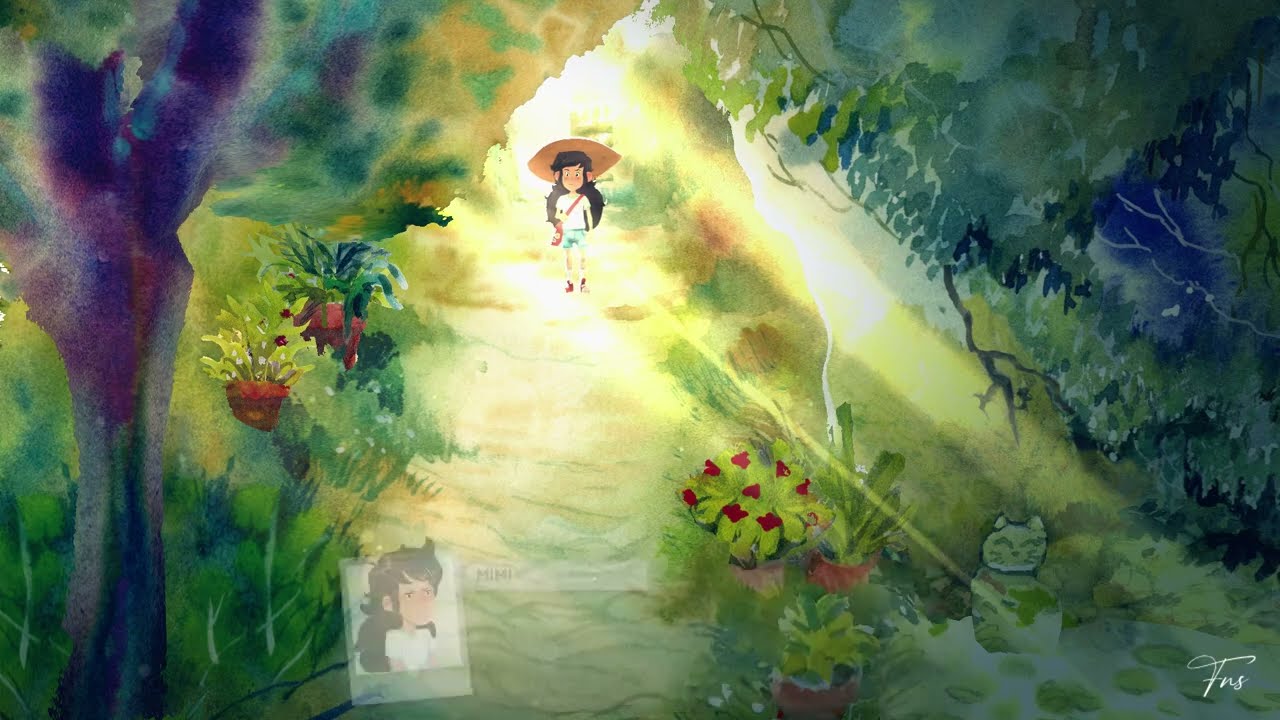The image is a vivid and lush representation of Japanese art in an anime or watercolor style. It portrays a dreamy garden scene with impressionistic and vibrant use of colors. Dominating the upper center of the image, a cartoonish girl stands illuminated by beams of sunlight. She wears a white shirt, blue shorts, red sneakers, and an extremely wide-brimmed hat, with a brown purse strapped across her shoulder, and she gazes forward, adding a focal point to the composition. 

The garden around her is lush with deep purples, blues, and greens. On the far left foreground, a uniquely colored tree painted in shades of purple, blue, maroon, and lavender stands out, blending into the green vegetation dotted with bursts of red flowers and other fauna. 

In the bottom portion of the image, slightly to the left, there is a nearly transparent portrait of a young girl or woman, perhaps a Polaroid, with a speech bubble next to it that says "Mimi." Towards the right, the greenery shifts to deeper hues of blue and black, with sunlight streaming through the trees in a streak of yellow, adding a touch of realism. A green cat is whimsically nestled among the foliage on the lower right-hand side, next to a cursive signature "FNS," likely the artist's mark.

Terracotta pots with plants are scattered amidst the flora, adding to the picturesque and cultivated atmosphere of the garden. All these elements weave together to form a captivating narrative, evoking the familiar motifs of anime while showcasing the artist's unique and expressive style.